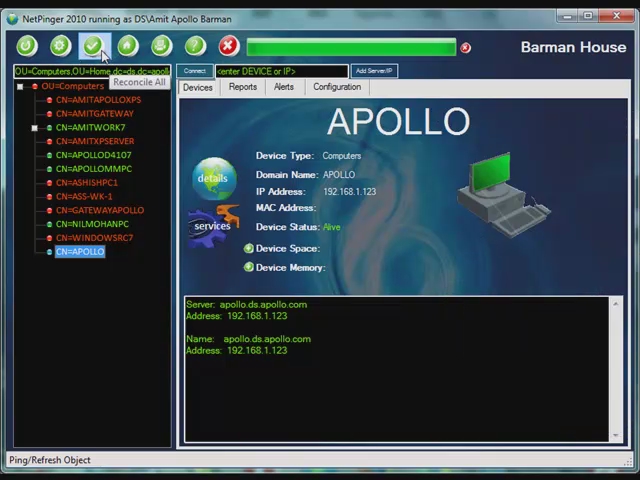The image depicts a computer monitor displaying a screenshot of a network management tool, identified as NetPinger 2010 running as DS Emmett/Apollo Barman. The interface features a navigation bar across the top with a blue and green globe icon, and various control buttons including a red "X", white square, and dash on a gray background. Below the navigation bar, the title "Apollo" is prominently displayed in white letters on a blue background.

The main section of the screen lists detailed device information in black text, with headers such as device type, domain name "Apollo", IP address (192.168.1.123), MAC address, device status (alive, highlighted in green), device space, and device memory. 

On the left side, there is a column containing bullet points and lists with items in red and green. The interface includes action buttons—green buttons with icons such as an arrow in a circle, a settings gear, a checkmark, a home, a printer, and a question mark, as well as a red button with a white "X".

Additional elements include a small green computer monitor icon, and various sections indicating 'Services' with a red and blue gear icon. The bottom section has text reading "ping/refresh object" in black letters on a white background. Overall, the screen displays a structured layout of network device details, statuses, and available actions for monitoring and configuration.